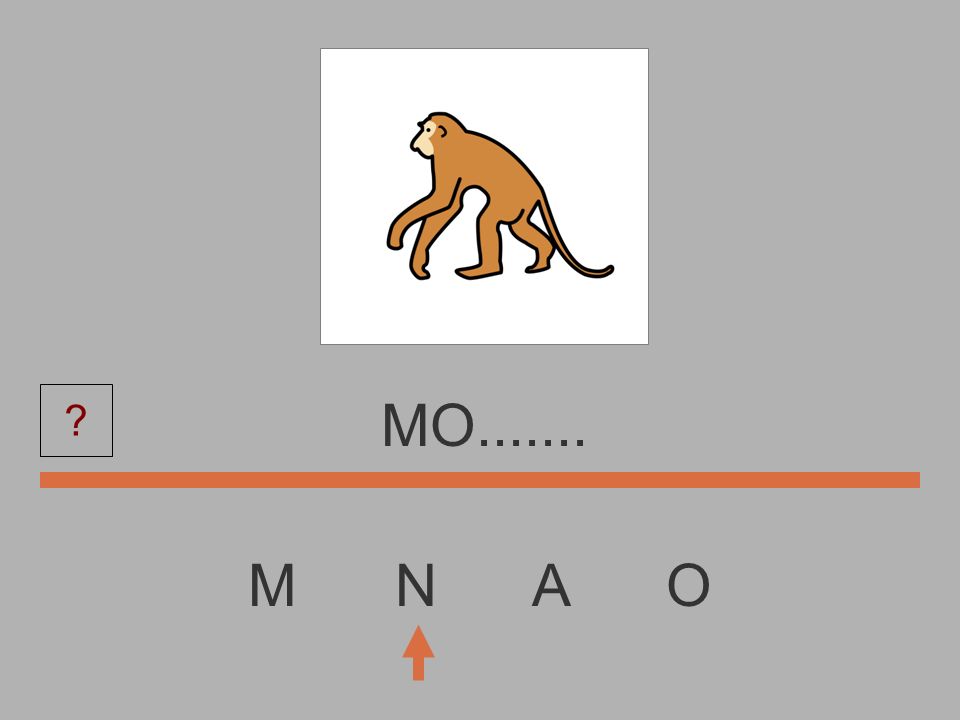The image features a digitally synthesized scene with a dark gray background. Centrally positioned near the top is a white square containing a cartoon drawing of a brown monkey with a lighter beige face, seen from a side view. The monkey is depicted walking on its hind legs while its forelegs touch the ground, and its long tail extends to the right. Below this square is a horizontal orange bar, and atop this bar, the letters "M O" are displayed in large black font followed by a series of ellipses ("..."), suggesting that more letters will follow. To the left side of the bar, there's a black-outlined square with a small red question mark inside. Directly beneath the orange bar, centered in the image, are the black letters "M N A O," each spaced apart. At the very bottom, aligned under the letter "N," an orange arrow points upwards, indicating a possible hint or direction towards the letter "N." Overall, the scene suggests an educational, perhaps spelling-related, exercise.